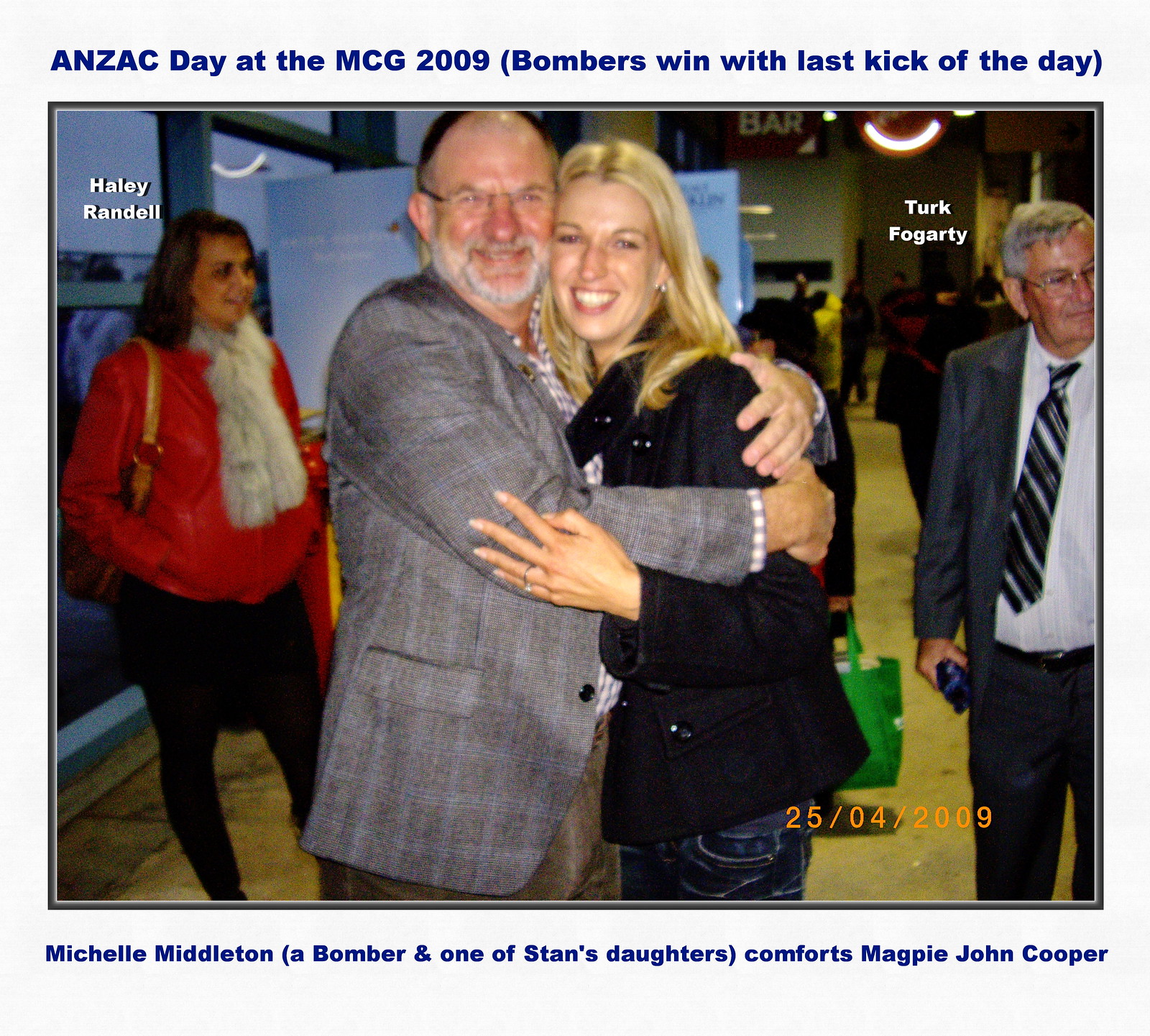In the center of the photo, an older man wearing a gray sports jacket and glasses is hugging a younger female with blonde hair, dressed in a black jacket and jeans. To the left of them stands a lady with brown hair, wearing a red jacket and gray scarf, with a purse over her shoulder; white letters above her head read "Haley Randall." To the right of the man hugging the young woman, there is another older gentleman in a suit and tie, with gray hair and glasses; above his head are white letters that say "Turk Fogarty." 

The background features a large glass wall, suggesting they are inside a convention center likely in the evening, given the dim light outside. In the lower right corner of the image, there is an orange date stamp that reads "25/04/2009." Below this date stamp is a caption in blue writing that says, "Michelle Middleton, a bomber, and one of Stan's daughters, Comfort's magpie, John Cooper."

Above the image, a title in blue reads "Anzac Day at the MCG 2009. Bombers win with the last kick of the day."